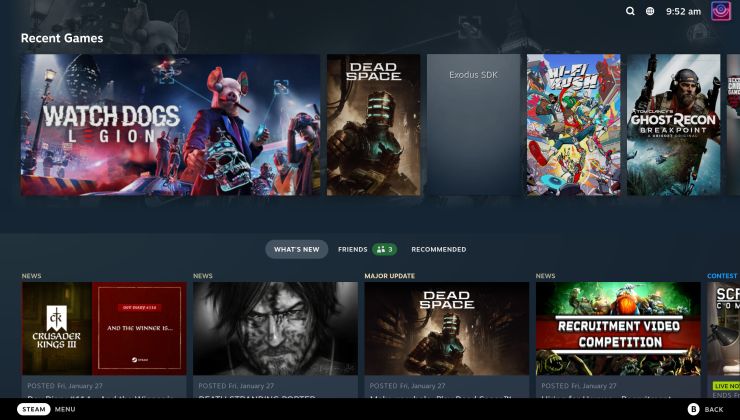The screen displays a dark charcoal-colored interface highlighting "Recent Games" on the left side. At the very top, there is a magnifying glass icon for searching, followed by a small unidentified icon, the time "9:52 AM," and then another colorful icon. 

Underneath the "Recent Games" section, the first game listed is "Watch Dogs: Legion," with "Legion" written in red and positioned below "Watch Dogs" in a wavy, underwater-like style. This section prominently features an image of a mouse puffing a cigar. 

Next is "Dead Space," showcasing robotic figures that evoke a sci-fi aesthetic. Following this is "Exodus SDK," which is depicted in gray, giving it a rather bland appearance. 

The next game, "Hi-Fi Rush," bursts with vibrant, cartoon-style graphics, presenting a lively and animated experience. "Ghost Recon Breakpoint" is also listed, featuring an illustration of a military figure, possibly airborne. 

Below these game titles, various interactive options are available under categories like "Possibilities," "What's New," "Friends Recommended," and "Major Updates," offering more choices for games the user might have played or be interested in discovering.